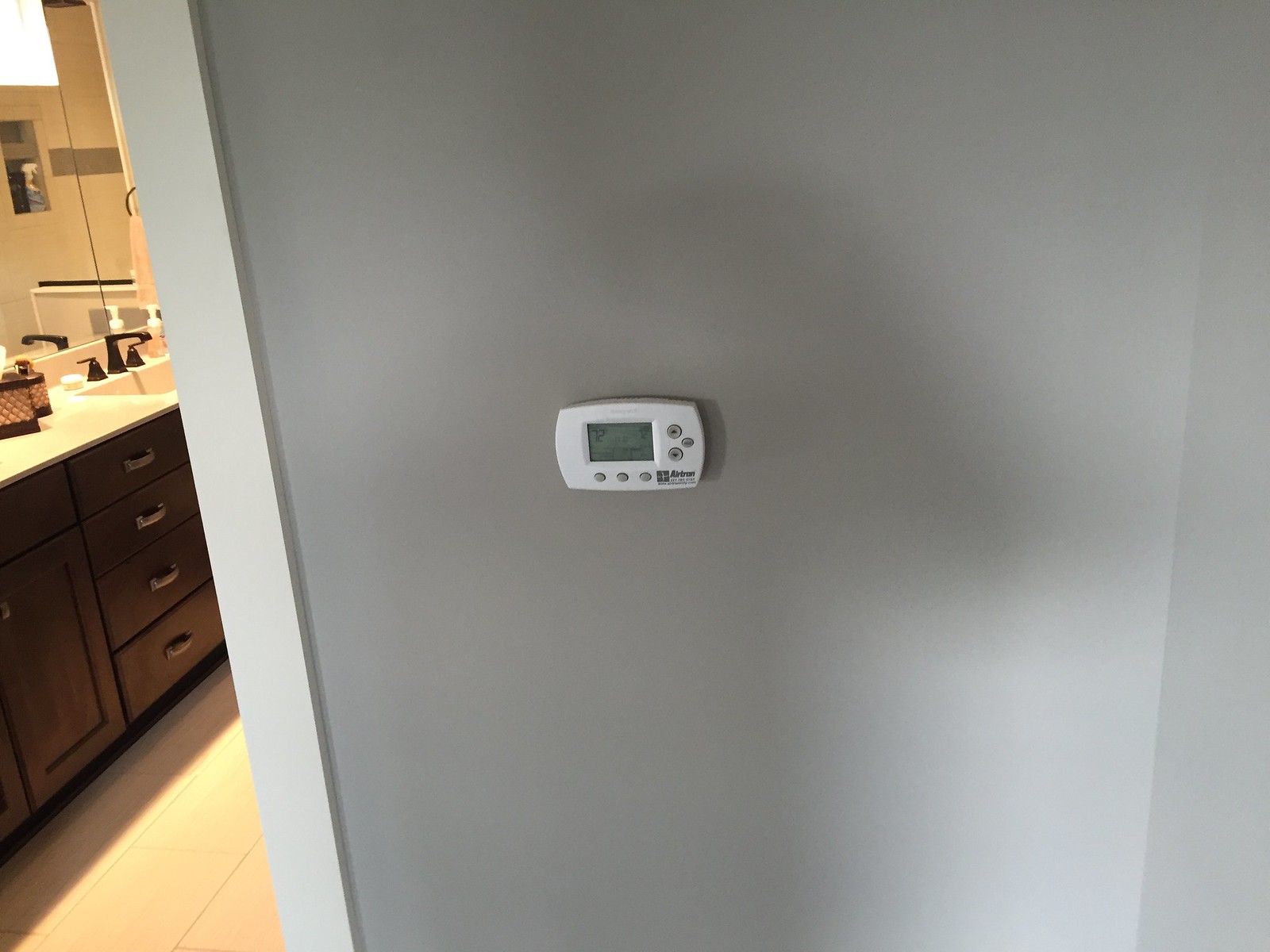The image showcases a light-colored wall adorned with a modern, white thermostat. The thermostat features a small screen displaying the temperature as 72 degrees. Below this screen, there are three oval-shaped gray buttons. To the right of the screen, two circular gray buttons with up and down arrows are visible. A brand logo is located at the bottom right corner of the thermostat.

On the left side of the image, a white door frame reveals a glimpse into a bathroom. The bathroom floor is covered with white tiles and is illuminated by overhead lights, casting a soft yellow glow. Inside the bathroom, there are brown wooden cabinets with four drawers, positioned below a mirror. A sink is situated under the mirror, and on the white countertop, several brown and beige objects are arranged.